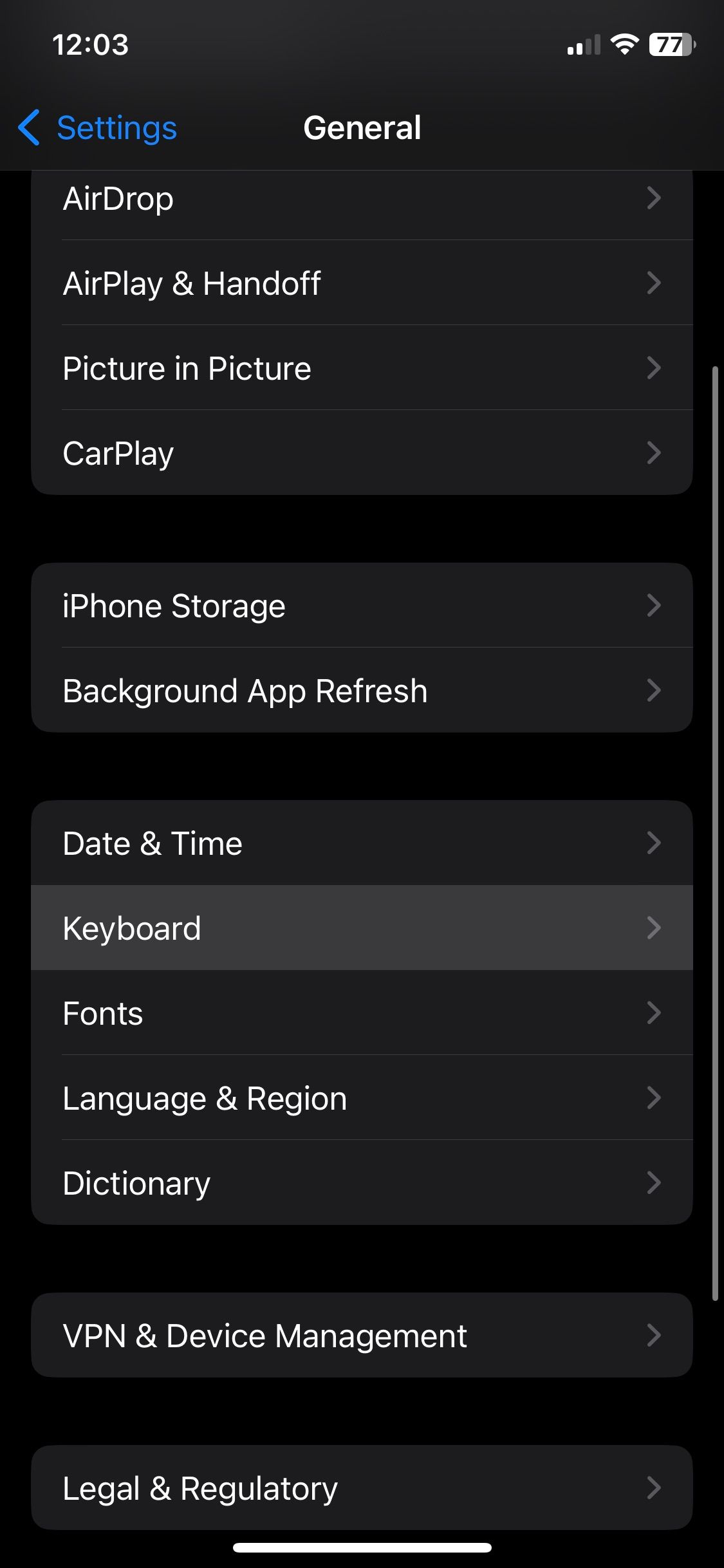A close-up image of an iPhone screen, displaying the Settings menu at 12:03 PM. The status bar at the top shows cellular data bars, Wi-Fi connectivity, and a battery life of 77%. The background is black, providing a stark contrast to the text and icons. At the top of the screen, "Settings" is highlighted in blue, the only splash of color. Beneath it, "General" is written in white text, indicating the selected category.

The menu is composed of several dark gray boxes, each containing different options. The first option is "AirDrop," followed by "AirPlay & Handoff." Next is "Picture in Picture," and then "CarPlay." There is a noticeable black space before the options "iPhone Storage" and "Background App Refresh."

Another black area separates these from "Date & Time," "Keyboard," "Fonts," "Language & Region," and "Dictionary." The "Keyboard" option stands out in a lighter gray, indicating it is currently selected. Beneath "Dictionary" is another black area, followed by "VPN & Device Management," with a final black space leading to "Legal & Regulatory." Each option features a right-pointing arrow (>) for navigation.